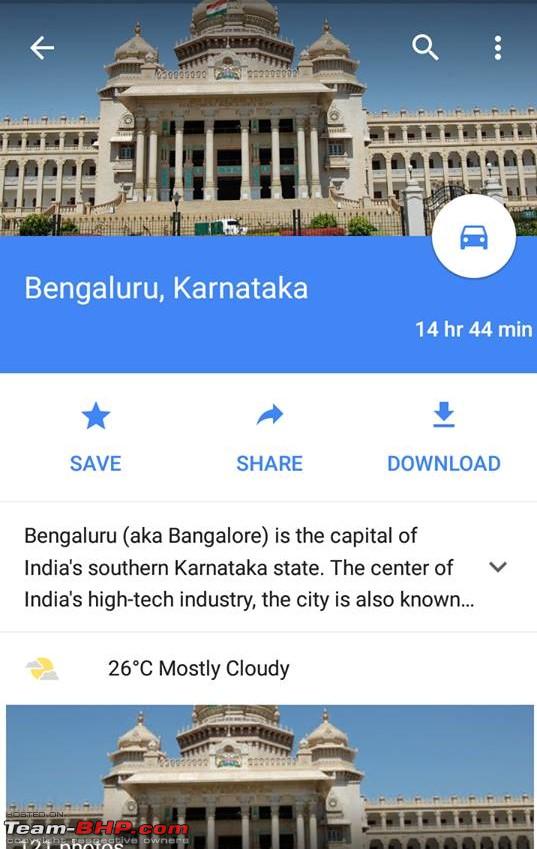Screenshot from a mobile phone showcasing a detailed interface likely related to a travel or mapping application. 

At the very top, the image features a photograph of a grand government building characterized by numerous archways and sections extending from the left and right. The central part of the building is a multi-storied structure with prominent pillars and large steps leading up to the entrance. Light blue banners are displayed around the entranceway.

In the top left corner of the screen, an arrow points to the left, while to the right, there is a white magnifying glass icon and three vertically aligned circles.

Below the photograph, a section with a light blue background reads "Bengalurakarnataka" in white text. Adjacent to this, a white circle contains a blue silhouette of a car, with the text "14HR44MIN" in white underneath.

Directly beneath this, three light blue buttons are labeled "Save," "Share," and "Download."

Further down, there's a text section with information about Bengaluru (Bangalore), describing it as the capital of Karnataka and the center of India's high-tech industry. Next to this text, an arrow points downwards.

Located below this, the weather information is displayed: "26°C, mostly cloudy" in black text, alongside a yellow sun icon partially obscured by gray clouds.

At the bottom, another photograph mirroring the top image of the government building is shown. The bottom left corner has the text "teambhp.com" and "121 photos," although this text is partially cropped.

This comprehensive caption meticulously details the content and layout of the mobile phone screenshot, providing a clear and vivid description for readers.